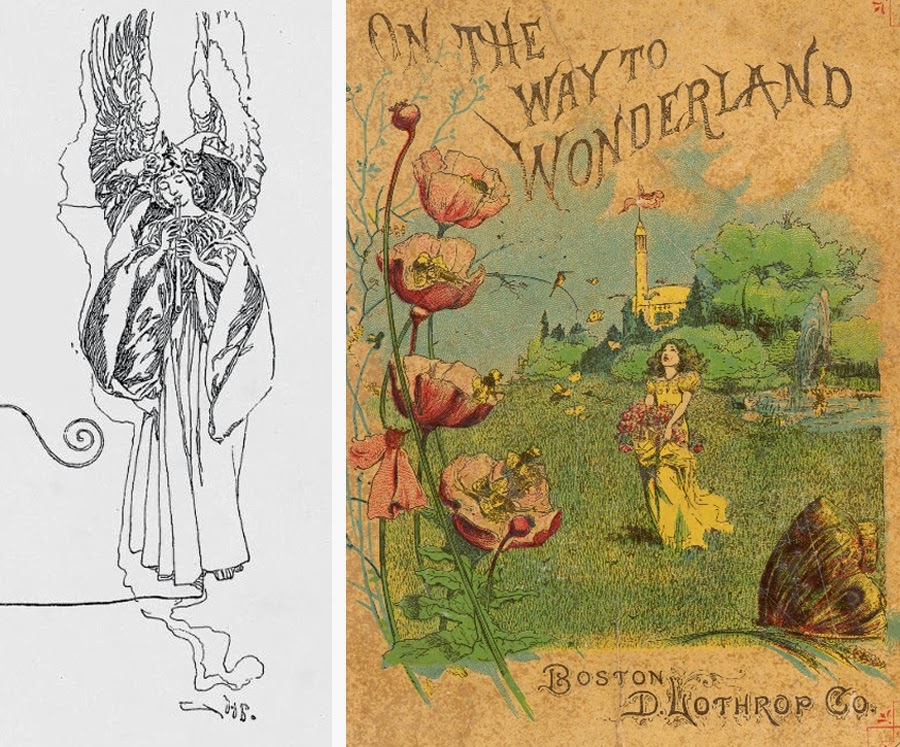This image is divided into two distinct parts. 

On the left, a black-and-white sketch drawn in either pen or pencil depicts an angelic figure. The angel, adorned in a long, flowing gown, appears to be playing a flute that remarkably has wings. The figure also wears a detailed headpiece that resembles leaves. The angel’s wings extend straight upward, and the sketch includes intricate details such as curly lines suggestive of smoke or mist at the base of the gown.

On the right, a vintage hand-painted poster features the title "On the Way to Wonderland" in bold, uppercase letters. Beneath the title, the text "Boston D. Hothrop Co." is visible. The scene illustrates a young girl in a bright yellow dress with puffed sleeves, holding red flowers amid a lush green forest. Her dark, curly hair cascades down as she gazes towards the title. Surrounding her are vividly colored red and pink flowers with yellow centers, set against an orangish and greenish background. In the distance, a yellow building resembling a church or castle with a flag is visible, along with a pond, trees, and distant birds. The entire right side has an old-fashioned, almost sepia-toned quality, enhancing its nostalgic and whimsical aura.